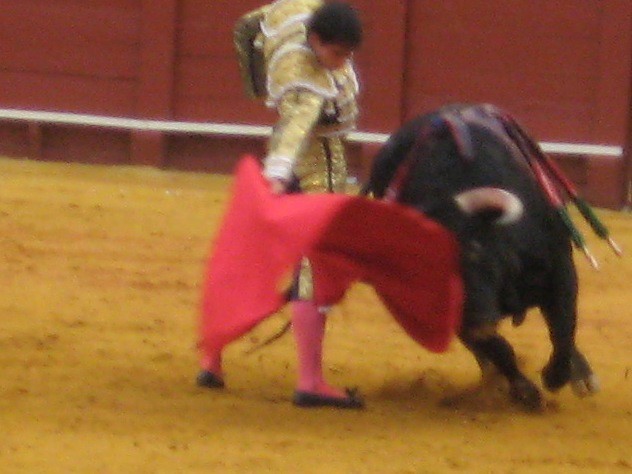The image depicts an outdoor bullfight in a large arena, featuring a traditionally dressed matador and a charging black bull. The matador stands centrally, clad in an ornate gold costume with big shoulders, pattern details, and matching gold pants. He also wears pink socks and flat black shoes. Wielding a red cape, the matador skillfully antagonizes the bull, which is mid-charge, its horns aimed directly at the red cloth. The ground beneath them is a yellowish-brown dirt, lending authenticity to the traditional setting. In the background, a solid red wall with a white horizontal stripe near its base runs across the top portion of the image, along with a white pipe or railing visible just above it. The scene, captured mid-day, emphasizes the dramatic interaction between the man and beast, set against vivid colors and a clear view of the arena's features.